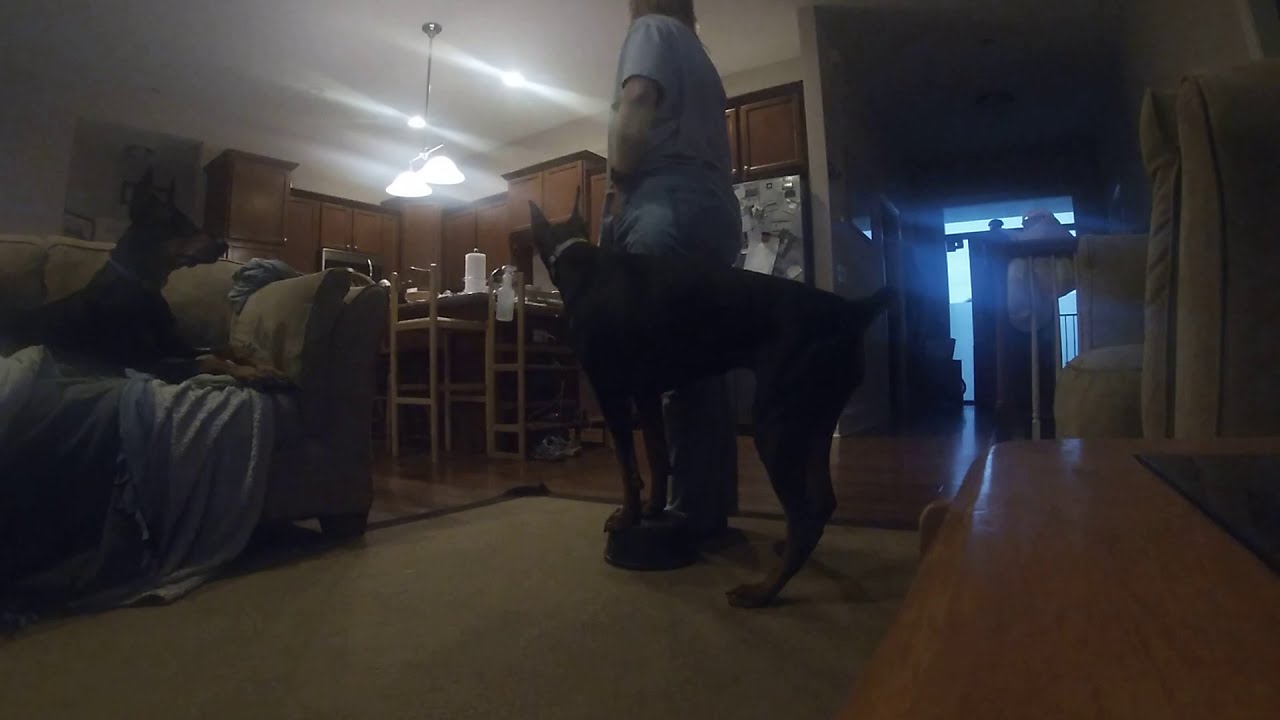In this dimly lit indoor setting, we're looking from near ground level towards a kitchen area illuminated by two overhead lights. Two Doberman Pinschers, identifiable by their distinctive black coats, pointy ears, and short tails, are the focal point. One Doberman is standing with its front paws on a pedestal, beside a person dressed in blue jeans and a gray shirt, possibly awaiting mealtime. The other Doberman is laying on a beige couch draped with a blue blanket, attentively observing the person. The backdrop showcases a kitchen with dark brown cabinets and a bar flanked by a few bar stools. The floor features a mix of hardwood and brown carpeting, adding warmth to the scene. In the background, there's a hint of blue sky visible through what could be a large window or doorway, contributing to the room's sparse lighting. The ambience suggests a cozy, everyday moment shared between the dogs and their owner.